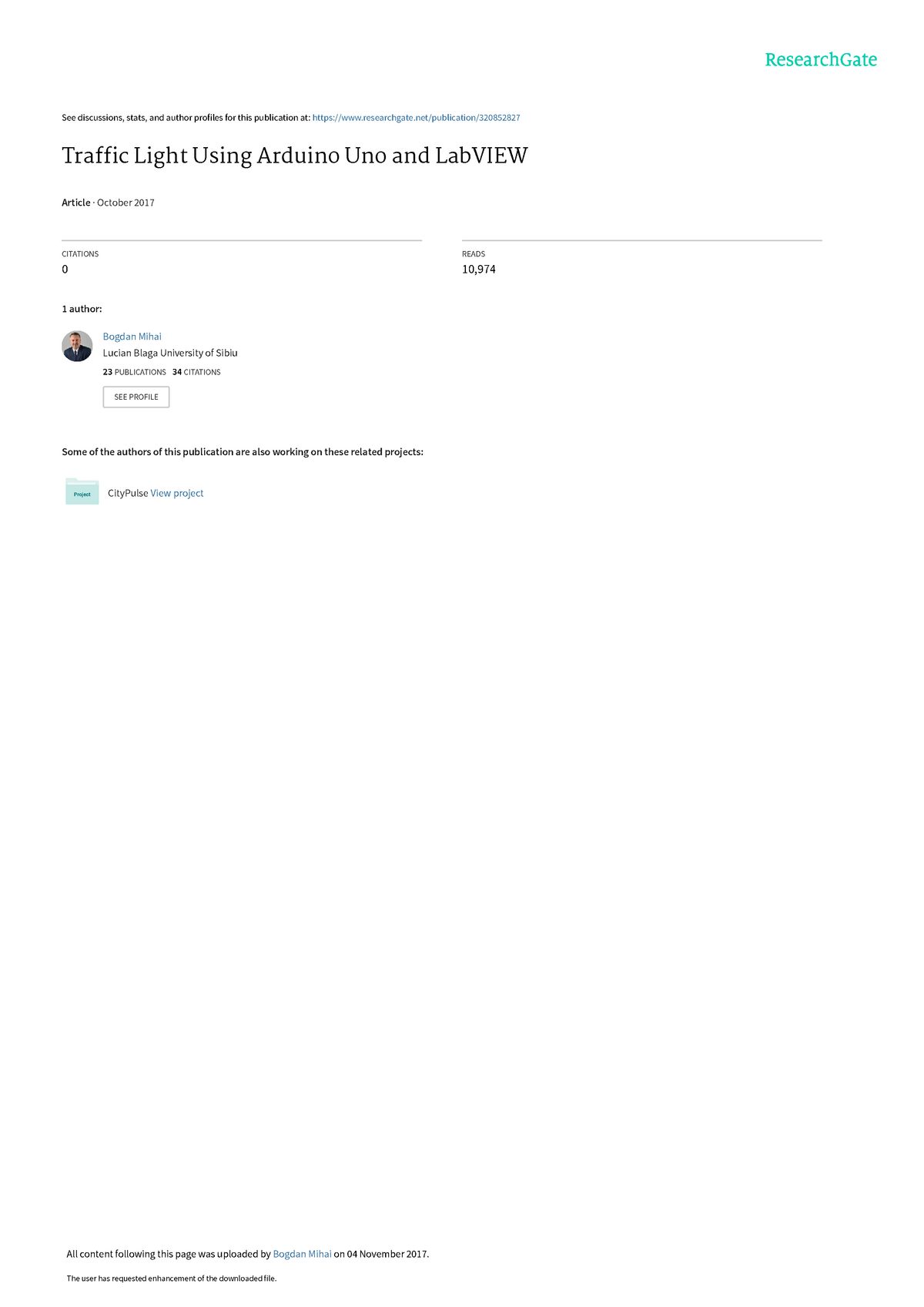Screenshot of an academic paper upload on ResearchGate. The top right corner features the ResearchGate logo in light blue letters, accompanied by a diminutive black sentence that includes a hyperlinked website also in light blue. Centered below this is the paper's title, "Traffic Light using Arduino UNO and LabVIEW," prominently bolded in black font. The next line details the paper's type and publication date, followed by the author's section on the left side, displaying his profile picture, name, and employment information with a "See Profile" button beneath. To the right, the number of views the paper has received is shown. Lower down, there's text prompting users to access more of the author's works. The overall backdrop for this screenshot is white, with all text rendered in a compact font. At the very bottom left, there's an additional line of small black writing coupled with a blue hyperlink.